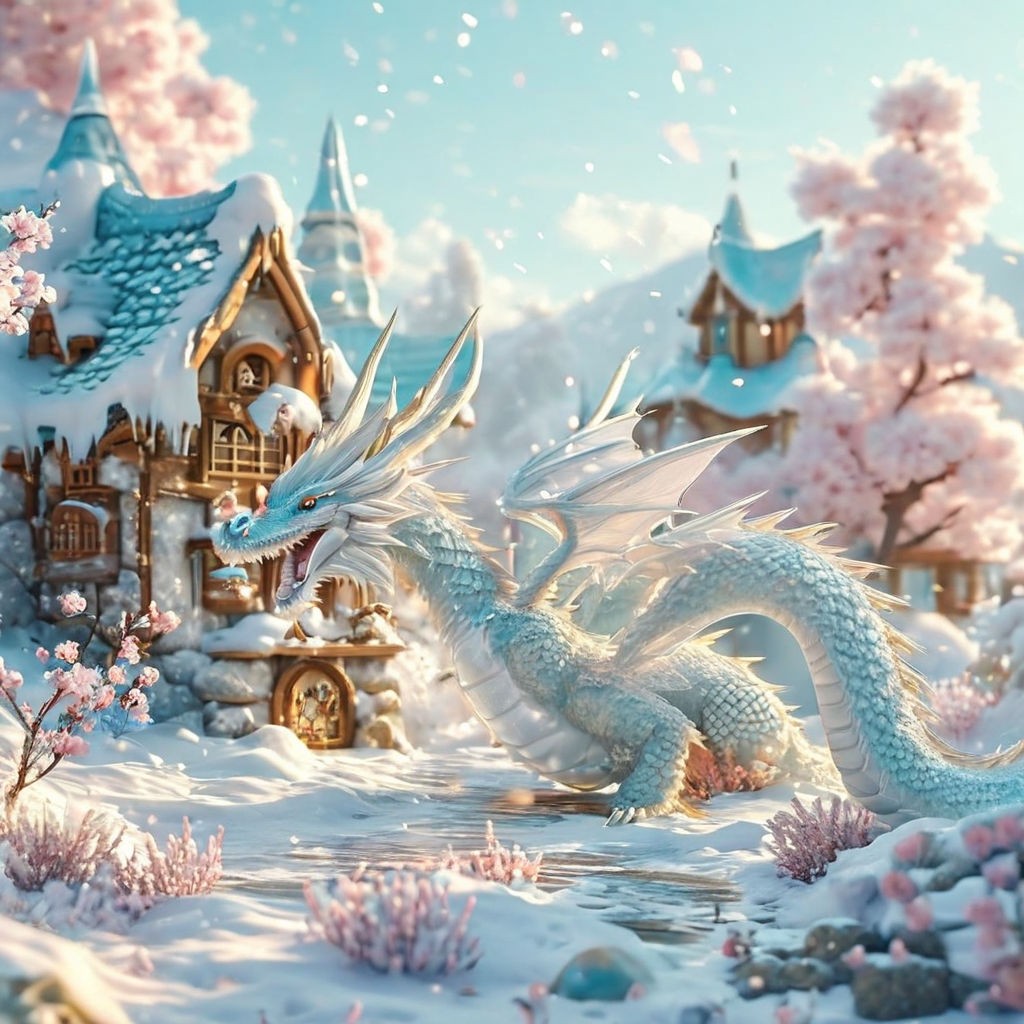This vibrant square image, measuring approximately six inches in height and width, presents a captivating scene set in a snowy, fantastical landscape that appears to be a painting or a computer-generated render. Dominating the right-hand side is a majestic ice or snow dragon, oriented towards the left. This striking creature features blue scales and a white underbelly, with wings of a whitish hue, adorned with a line of spikes down its tail and prominent horns on its head. Its piercing golden-amber eyes stand out against its frigid palette.

In the foreground, a snow-blanketed courtyard is dotted with tufts of resilient pink flowers and delicate brown branches also in bloom with pink petals, offering a splash of color amidst the wintry setting. Beyond the dragon, the background boasts quaint, older country-style arched buildings, characterized by sturdy wooden doors and frames, along with shingled blue roofs laden with snow.

The tranquil sky above is a serene light blue, speckled with soft, white clouds, which add to the overall calmness of the scene. Encompassing the landscape are trees adorned with plush, pink foliage, creating an enchanting and otherworldly atmosphere.